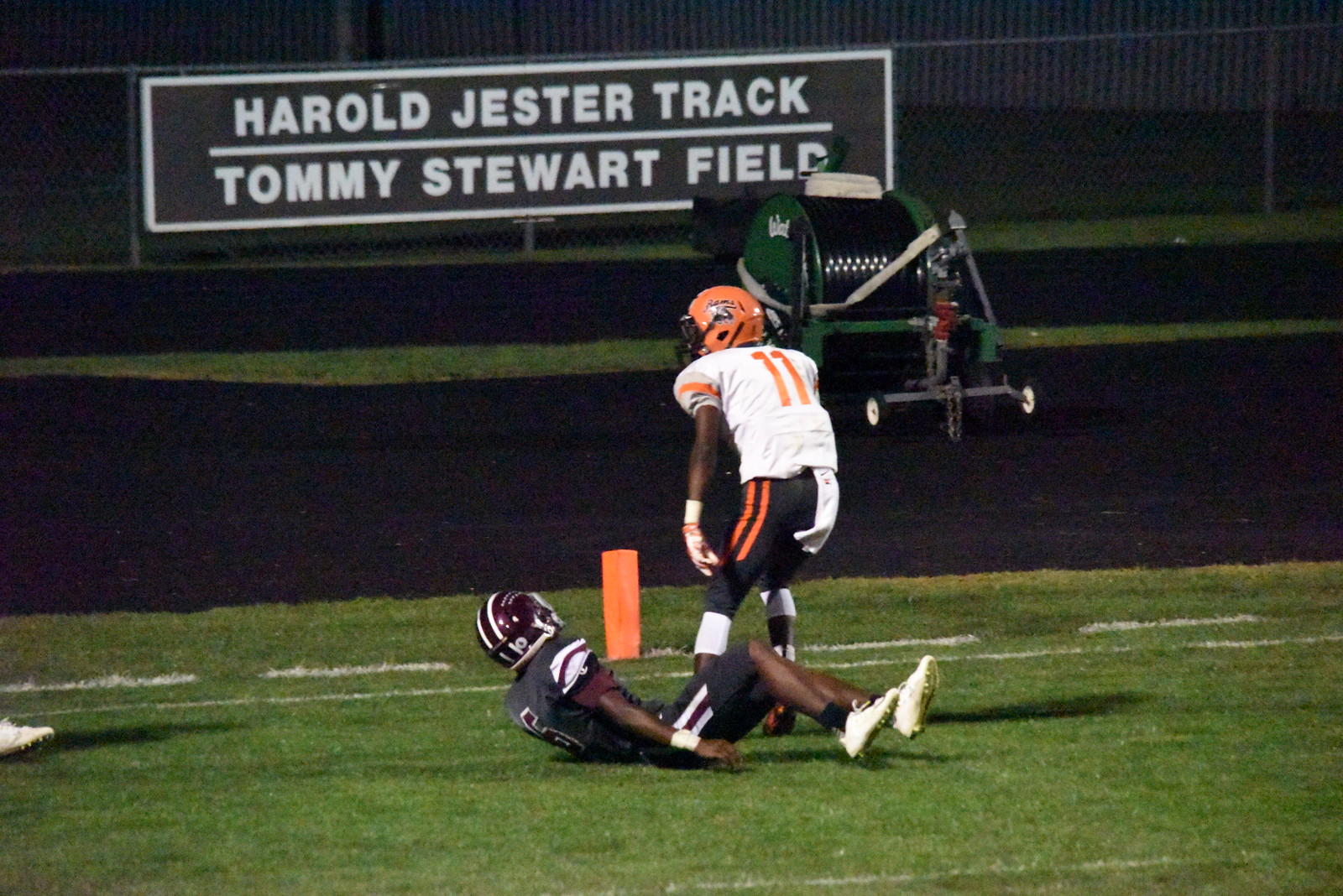This photograph captures a nighttime American football game, featuring two players on what appears to be a college-level field. The background is dimly lit, with the green grass of the illuminated field standing out against the dark surroundings. White yard markings demarcate the playing surface. A distinct chain-link fence lines the back of the scene, where a sign with white lettering reads "Harold Jester Track, Tommy Stewart Field."

In the image, the central action involves two players with dark brown skin. One player is standing and dressed in a white jersey with the number 11, black pants marked with orange stripes, and an orange helmet. His opponent lies on the ground, sporting a black outfit with white and maroon stripes and a brownish, maroon-like helmet with white stripes. Both players wear white cleats. An additional white cleat from another player is visible at the bottom left of the image. An orange yard marker further defines the scene, highlighting the intensity and detail of this well-lit, competitive moment on the field.